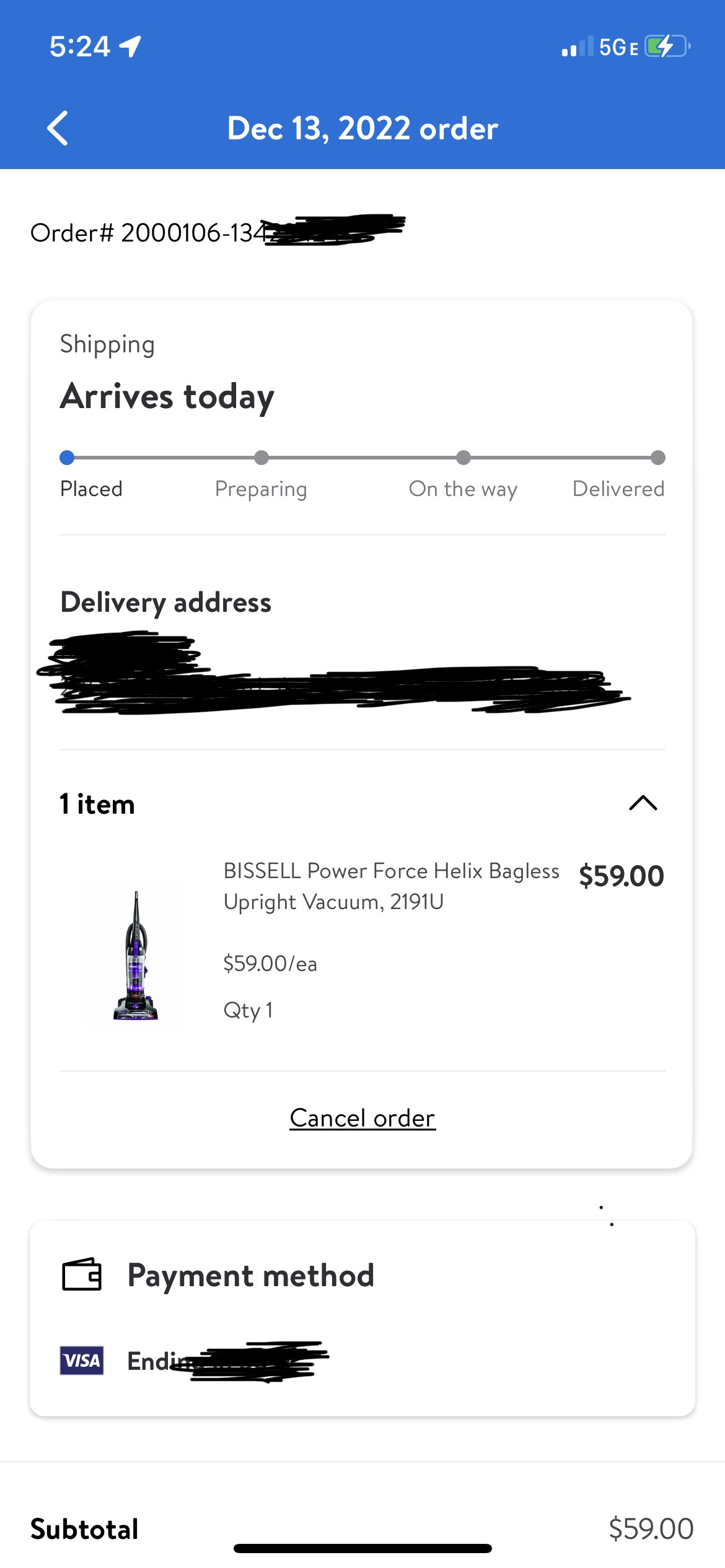This image appears to be a screenshot from a mobile device, possibly a cell phone or tablet. The top status bar displays the time "5:24" in the upper left corner, an upward-pointing arrow (indicating upload or signal direction) towards the northeast, a "5GE" and two signal bars indicating the network strength, and a battery icon with a charge symbol. The bar at the top is highlighted in blue.

Centrally placed within this bar is the date "December 13, 2022," followed by the word "order," suggesting an order tracking screen. Directly below this, the text "order number" is visible alongside the partially obscured order number "2106-134," with the rest redacted for privacy.

Next, a section titled "Shipping" indicates that the arrival is scheduled for today. Below this, a progress bar for the order status is depicted, with stages labeled as "Placed," "Preparing," "On the way," and "Delivered." The current status shows as "Unplaced."

Further down, there's a title "Delivery Address," but the actual address has been scribbled out to maintain privacy. Underneath, there is a listing for one item: a "Bissell Power Force Helix Bagless Upright Vacuum 2191U" priced at $59.00 each, with a quantity of one, and an option to "Cancel order."

Finally, at the bottom, a "Payment Method" section is shown, where the payment was made via a Visa card, though the card details are scratched out for security. The subtotal of the order is noted as $59.00.